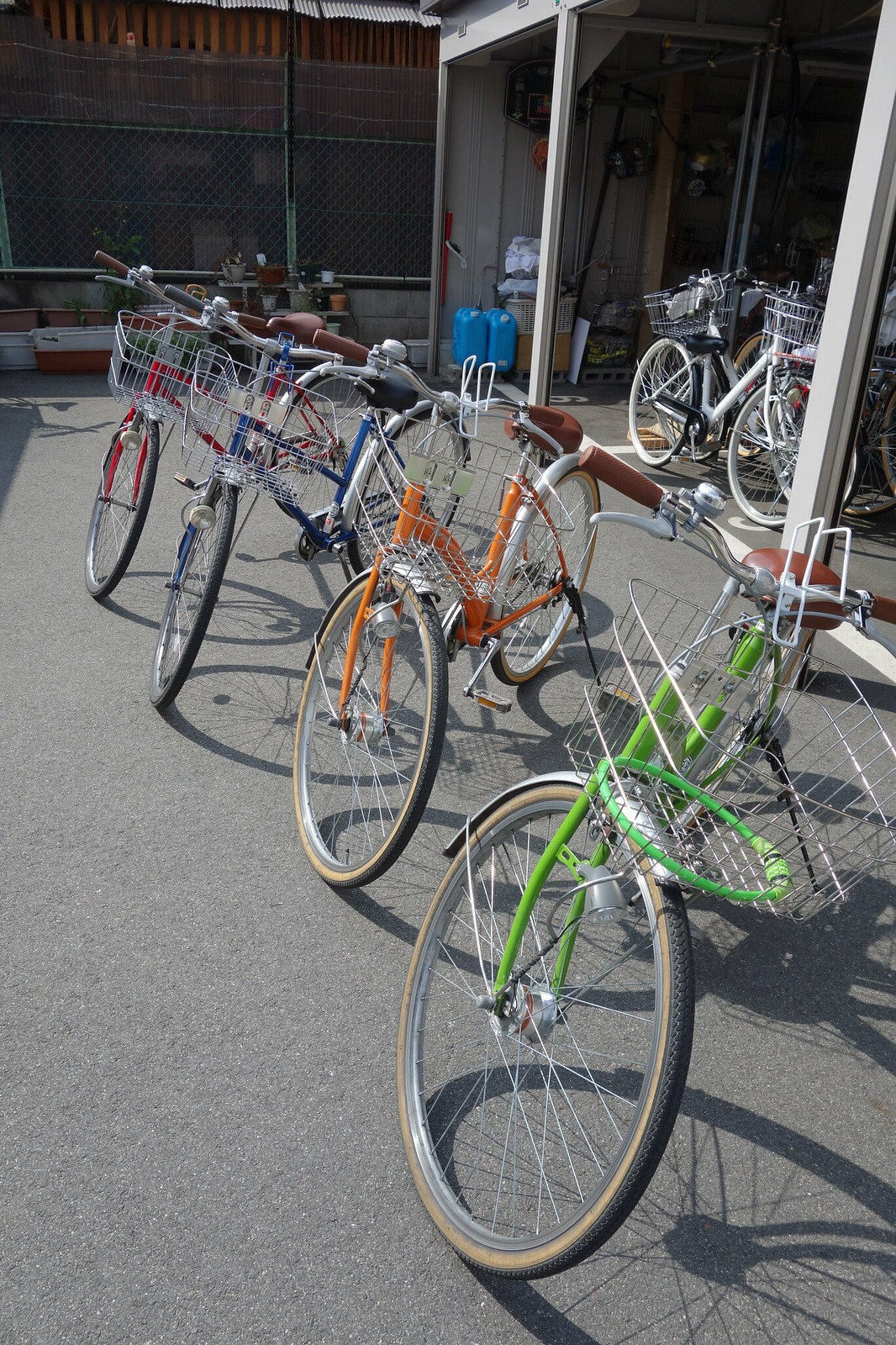This photograph depicts a somewhat run-down cement area adjacent to a building and under an overhang resembling a carport or garage. Arranged diagonally from the top left to the bottom right of the image, four distinctively colored bicycles—red, blue, orange, and green—are parked with their front wheels angled to the left. Each bike is equipped with a basket either in the front or at the back. Behind these bicycles, wooden two-by-fours support a roofing structure under which additional bikes are visible. The background features a high wooden fence towards the upper back left corner of the image, and a garage with open doors exposes various items such as gas cans and a laundry hamper. Shadows from the bikes cast onto the ground, indicating it's a sunny day. Despite a discrepancy in reported colors for the first four bikes and one purple bike, the dominant consensus is on the specific arrangement and setting, with the main focus on the colorful bikes lined up on the cemented pavement.